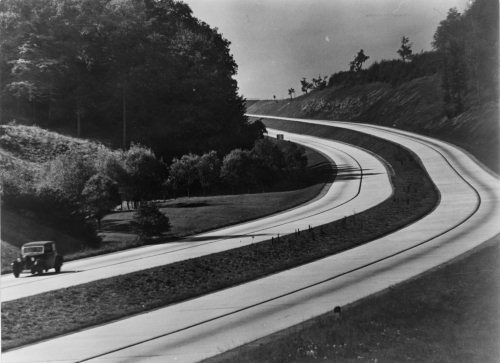This horizontally oriented black and white photograph, seemingly from the 1940s to the 1960s, captures a tranquil scene of a dual-lane road cutting through a valley during daytime under a light gray, possibly cloudy sky. The image appears to be taken from an elevated vantage point, potentially a hill, looking down on the scene. Dominating the landscape are two parallel roads, each with two lanes, separated by a grassy median. The roads curve gracefully in a backwards C-shape. 

On the left side of the image, a small hillside dotted with trees and shrubbery can be seen, while the right side also features hills with dispersed trees. The road lacks the modern dotted lane markings and instead is divided by a solid line. In the bottom left of the image, a lone black car, reminiscent of models from the 1930s to 1950s with its thin wheels and boxy yet slightly rounded shape, travels towards the left. The foreground is marked by short-cut grass and the overall scene is serene, emphasizing the era's simpler, less crowded roadways.